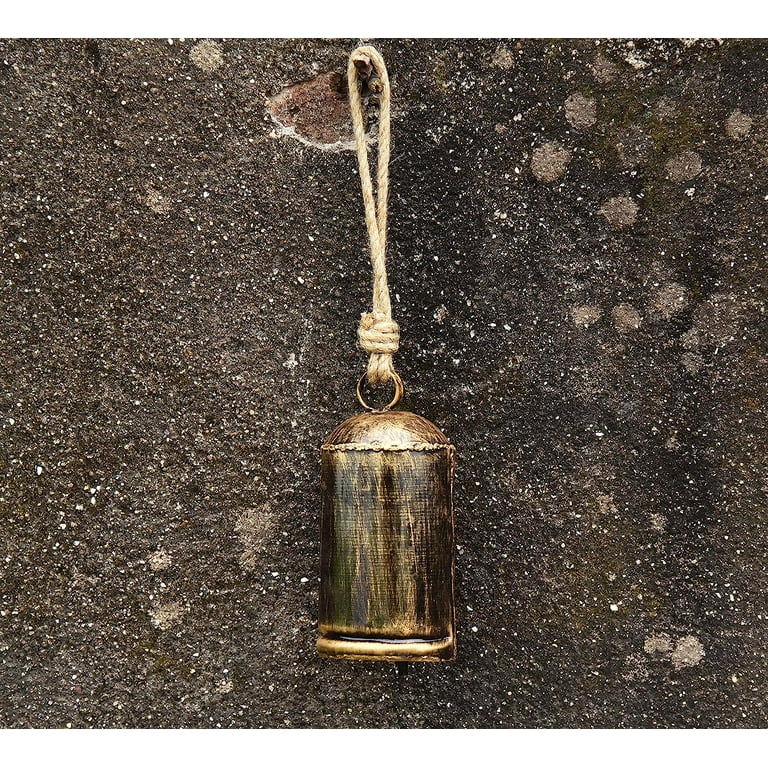This large square image features an antique-like ornament hanging from a wall composed of textured, dark brown stone with some light brown circular spots particularly visible in the upper right corner. At the top center of the image, a nail protrudes from the wall, from which dangles a piece of tan-colored twine. One end of this twine is tied to a small gold ring, which is attached to a cylindrical object with a domed top, resembling an old-style bell. The bell-like object, stained with dark brown and black hues, hangs centrally in the image. The overall composition gives the impression of a rustic, vintage setting.